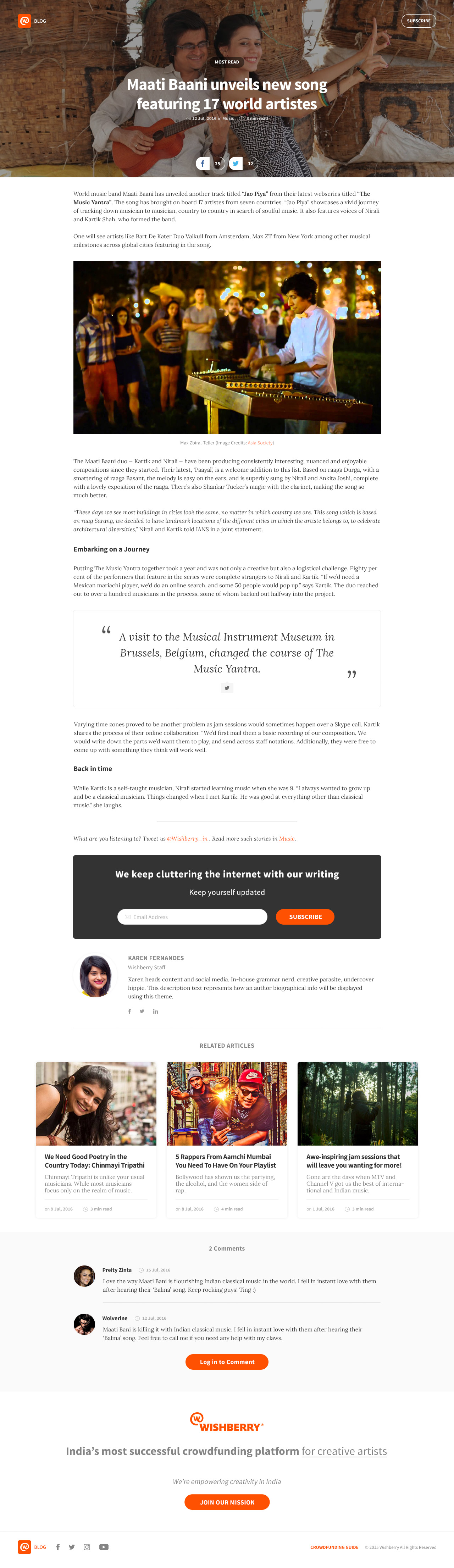**Caption:**

The image captures the top section of an extensive webpage featuring vibrant and engaging content. At the top, there is a colorful background photo showing two joyful individuals leaning against each other. On the left stands a man in a white shirt, beaming as he strums a small, vividly red guitar or ukulele-like instrument. Beside him, a woman wearing a black and white dotted dress is also smiling. She is striking playful poses with her fingers and has a rainbow band adorning her arm. Her long black hair is tied back, and she looks directly at the camera, exuding positivity.

Overlaying this image is prominent large white text announcing, "Matti Bani Unveils New Song Featuring 17 World Artists." Below this headline are two social media buttons—a Facebook logo on the left and a Twitter logo on the right.

Following the header, the webpage is composed of several paragraphs of text accompanied by various images and pop-out sections. After the first two paragraphs, there’s an image of a night scene depicting a group of people in the background observing a man playing a large stringed instrument laid out like a table in front of him. This musician, dressed in a white shirt with medium-length black hair, is illuminated by strings of lights around the gathering, enhancing the nocturnal ambiance.

As the content continues, a notable quote is presented within an image, stating, "A Visit to the Musical Instrument Museum in Brussels, Belgium Changed the Course of the Music Yantra," displayed in large quotation marks. This is followed by additional text leading to a black box with a message encouraging readers to stay informed: "We Keep Cluttering the Internet with Our Writing. Keep Yourself Updated." Below, there is a subscription bar featuring a field labeled "Email Address" and an adjacent bright orange "Subscribe" button inviting readers to join the mailing list.